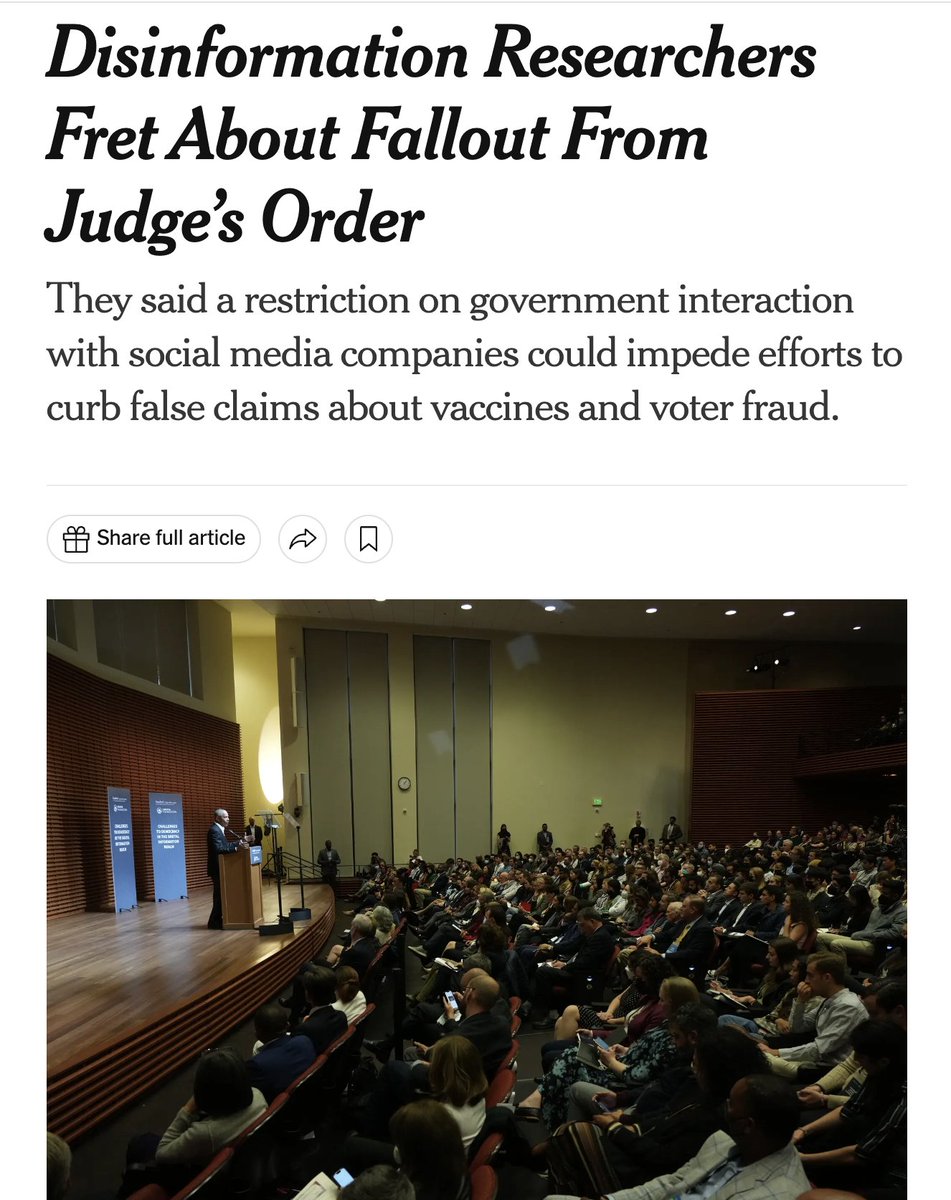A screenshot from a web article is depicted. The article appears to be hosted on a website where content can be shared and gifted. The headline reads: "Different Information Researchers Fret About Fallout from Judges’ Orders" in bold black text. Below the headline, a smaller caption states: "They set a restriction on government interaction with social media companies which could impede efforts to curb false claims about vaccines and voter fraud." 

Below this text, there is an icon representing a gift, enclosed in a circular box that indicates the option to "Share" the article. Adjacent to this is another circle containing an icon for bookmarking the article.

The image in the article shows several people seated in an auditorium-like setting, all facing towards the left side of the photo. They are focused on a man standing at a podium on a stage to their right. The man at the podium appears to be addressing the audience, and behind him are two whiteboards positioned on the stage.